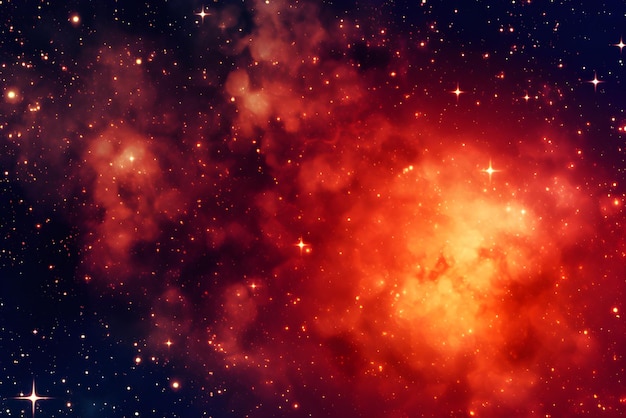This image presents a detailed and vibrant depiction of deep space, where a vast array of stars twinkles against a predominantly black canvas. Dominating the bottom right quadrant, there is a vivid, explosive glow that transitions from a central white to yellowish core, spilling outwards into deep reds and oranges, and then fades into a smoky translucence. This brilliant, starburst-like formation, possibly a nebula or an exploding star, extends its fiery tendrils towards the top middle and left of the image. Throughout this galactic scene, numerous stars of varying brightness and sizes punctuate the darkness, some even shaped like crosshairs or T-shapes. Their white and yellowish glows pierce through the translucent nebula dust, creating a mesmerizing interplay of light and color that highlights the dynamic and awe-inspiring beauty of the cosmos.